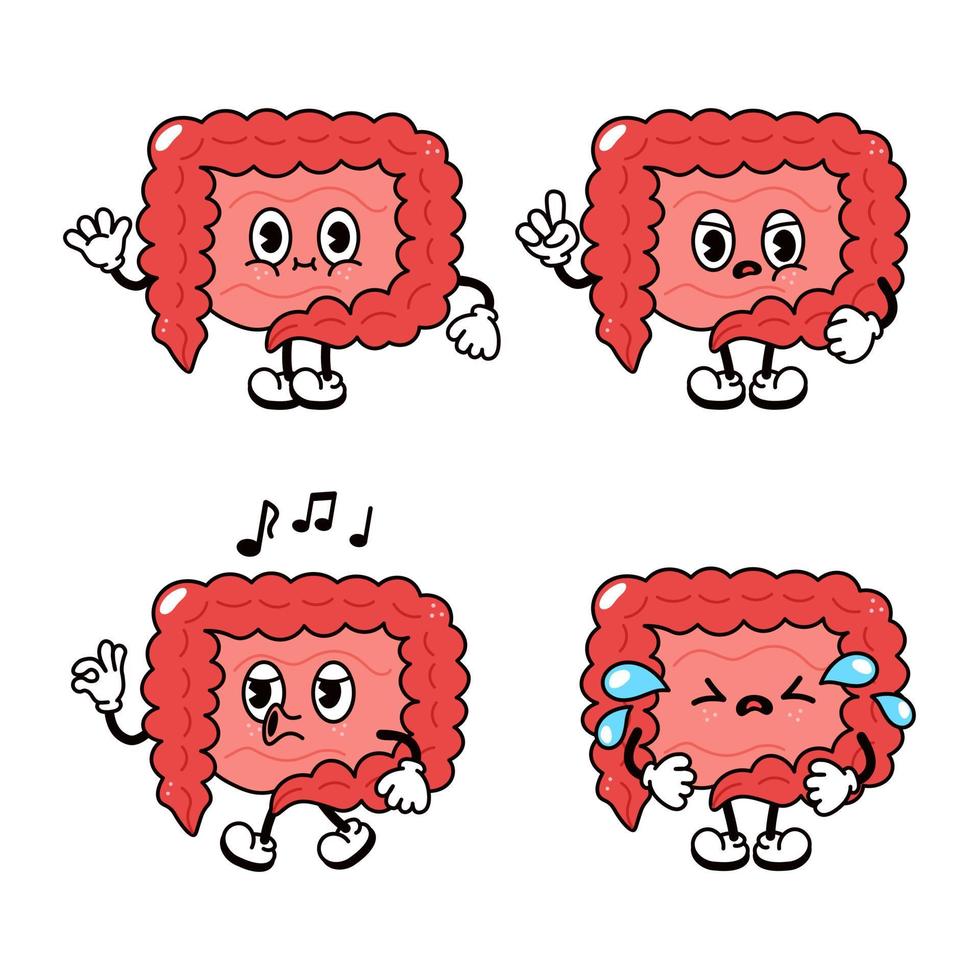The image is a four-panel cartoony poster of a single character, which appears to be an anthropomorphized square-shaped figure with peach and orange coral coloring. This character is quite unique with a puffy, not human form, featuring spindly legs wearing oversized white shoes reminiscent of the California Raisins. Its round eyes have endearing fat cheek lines underneath, and it dons white gloved hands also akin to California Raisin hands.

In the first top-left panel, the character is standing and looking straightforward. Moving to the top-right, its hand moves closer to its face, one finger pointed upwards as if to explain something, with eyes slightly droopier. The bottom-left panel shows the character with its right hand forming an A-OK sign, three musical notes above its head suggesting it is whistling or singing, its puckered mouth visible, and eyes still somewhat lidded. In the final bottom-right panel, the character appears frustrated, stomping its feet with squinted eyes and an expression indicative of crying with tears or sweat splashing away from its face. Notably, the character exhibits a range of emotions and actions across the panels, all set within a monochromatic pink palette aside from the blue tears.